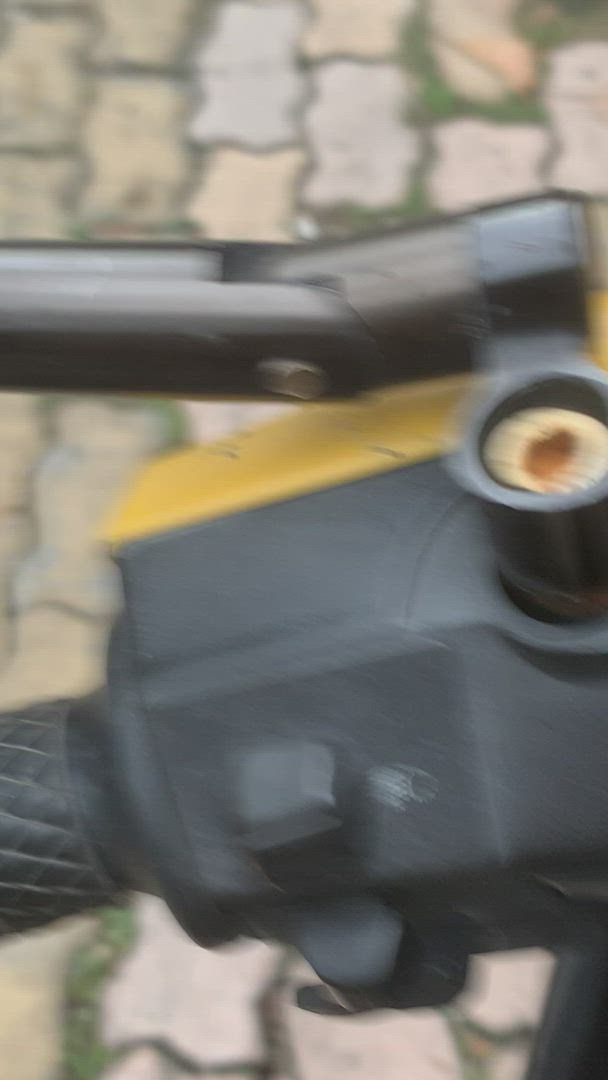A blurred photograph depicts the handlebars of what appears to be an electric bike against a backdrop of multicolored, irregularly shaped pavers. The bike's handlebars are predominantly black, featuring a yellow component at the front that includes a switch, likely indicating its electric functionality. The image captures the bike's brake levers positioned at the top, alongside a yellow element and a cylindrical piece with yellow detailing at the center. The handlebar, visible on the right side of the frame, suggests focused functionality, possibly including an electronic headlight switch, while the left side remains out of view. Below the handlebars, the ground's wavy-edged, multicolored paving stones add texture and depth to the scene.